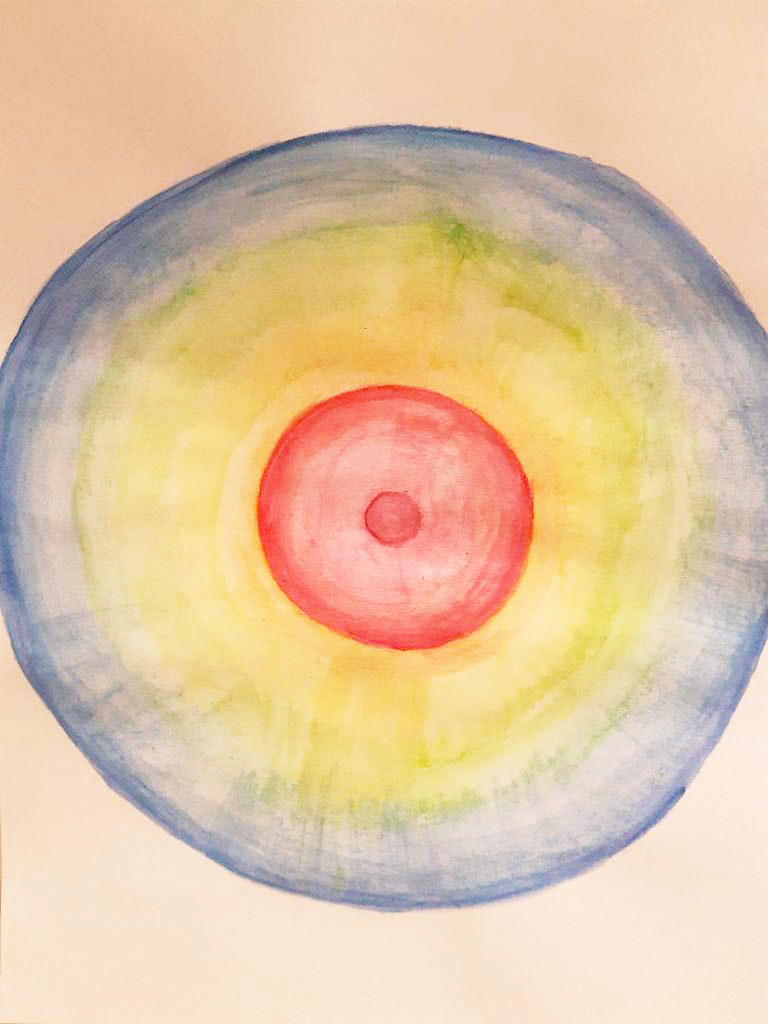The artwork appears to be a detailed representation of a bullseye rendered either in marker or watercolor. It features a circular bullseye prominently positioned in the center of a rectangular canvas with a pink background. The bullseye spans the entire width and almost the entire height of the canvas, leaving minimal pink space at the top and bottom edges.

Starting from the outermost edge, the bullseye begins with a dark blue ring that gradually fades into a lighter blue as it approaches the center. This blue gradient transitions into a very light green band, which further blends into a thicker yellow section. The yellow ring then fades to a prominent red circle at the core of the bullseye.

This red circle is distinctly outlined and darker near its border. An additional, smaller circle exists directly at the center of the bullseye, featuring a heavily shaded red border and an intensely red core. The overall composition creates a visually striking depiction of concentric circles with a dynamic color gradient effect.